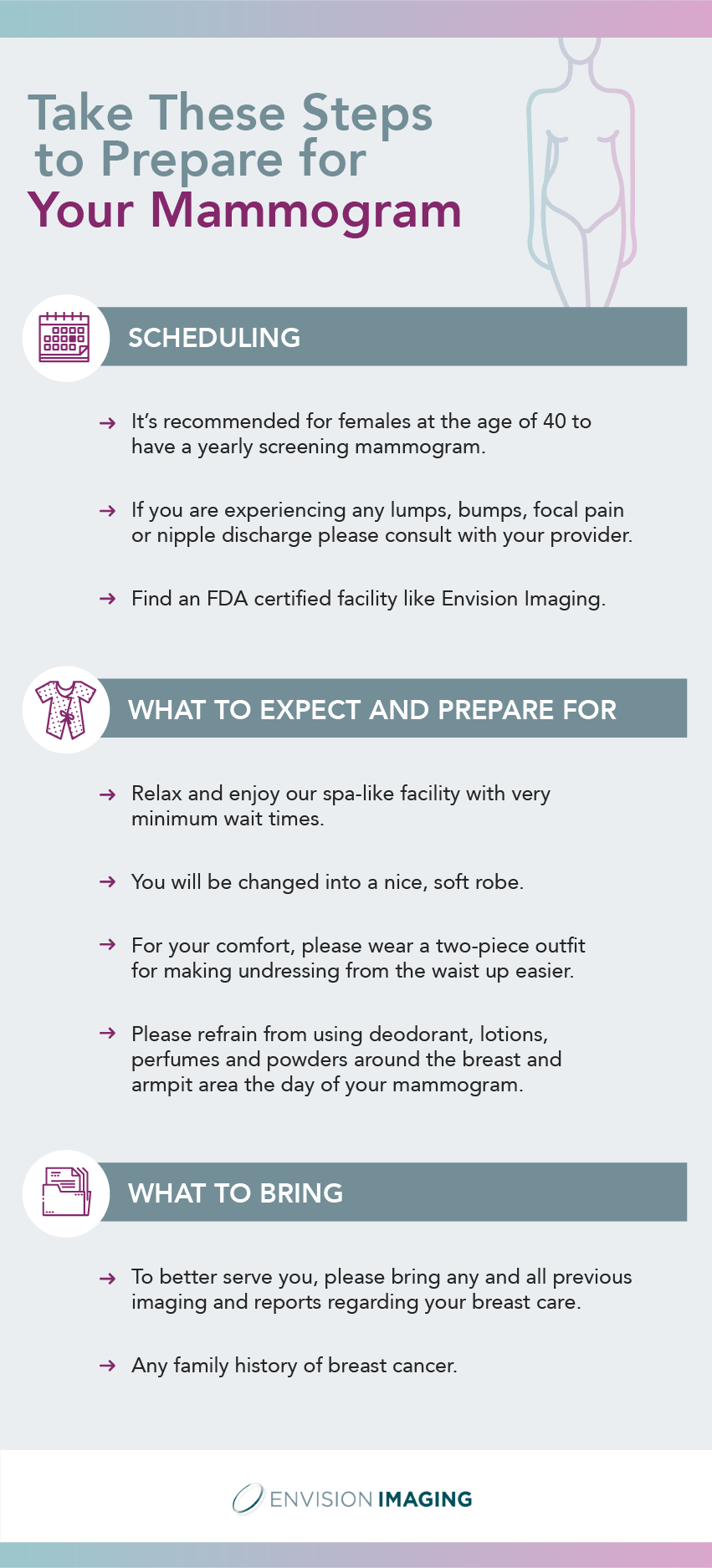The information brochure from Envision Imaging features a calm and soothing pastel palette, predominantly showcasing shades of turquoise, pinkish hues, and light blue, creating a mellow and clean aesthetic with a medical theme. The vertical layout is divided into three main sections, delineated by different hues of blue to purple gradients and soft colored lines.

At the top, the title "Take these steps to prepare for your mammogram" is prominently displayed in grey and purple. Below it, an outline of a woman's body lends an illustrative touch to the design.

The first section, "Scheduling," emphasizes the importance of annual mammograms for females aged 40 and above. It advises consulting a provider if experiencing symptoms such as lumps, pain, or nipple discharge, and recommends finding an FDA-certified facility like Envision Imaging.

The second section, "What to Expect and Prepare For," suggests a relaxing experience akin to a spa visit, where patients will change into a soft robe. Practical advice includes wearing a two-piece outfit for easy undressing and avoiding lotions, perfumes, and powders on the day of the mammogram.

The final section, "What to Bring," underscores the importance of bringing previous imaging, reports, and any family history of breast cancer to the appointment to ensure comprehensive care.

Overall, the infographic melds essential pre-mammogram instructions with a serene visual presentation, aimed at making the experience as comfortable and informative as possible.